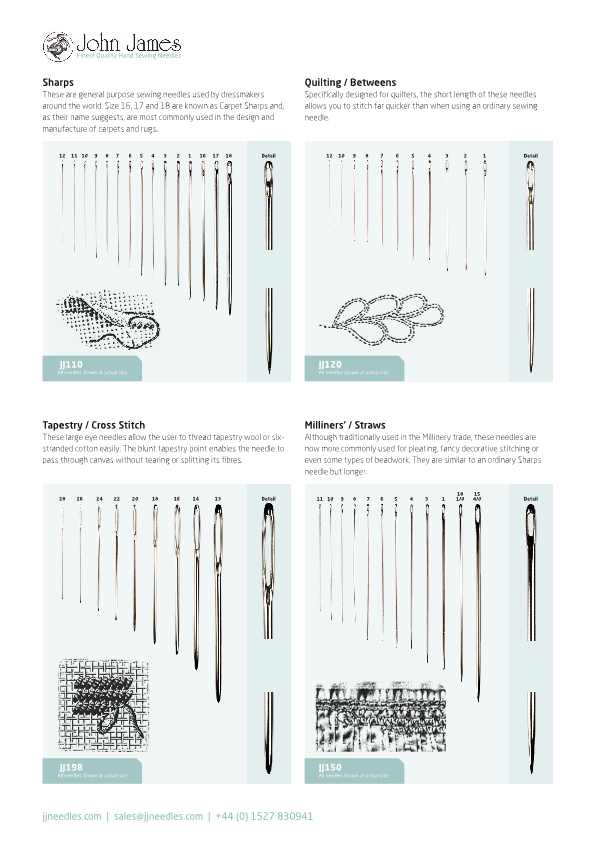This image is an advertisement for John James fine quality hand sewing needles. It is divided into four quadrants, each highlighting a different type of needle: "Sharps" (top left), "Quilting/Betweens" (top right), "Tapestry/Cross Stitch" (bottom left), and "Milliners/Straws" (bottom right). Each section features rows of needles arranged from smallest to largest, along with illustrations of the stitching patterns that can be achieved with these needles. The sections also include brief descriptive text and numbers, such as 110, 120, 150, and 198. The background of the photograph is lightly teal, set against a white paper backdrop. The name "John James" is prominently displayed in the upper left corner, indicating the brand, with additional branding text stating "fine quality hand sewing needles" and a logo. At the bottom of the image, there's a website (jjneedles.com) and a contact phone number (440-152-7830941).